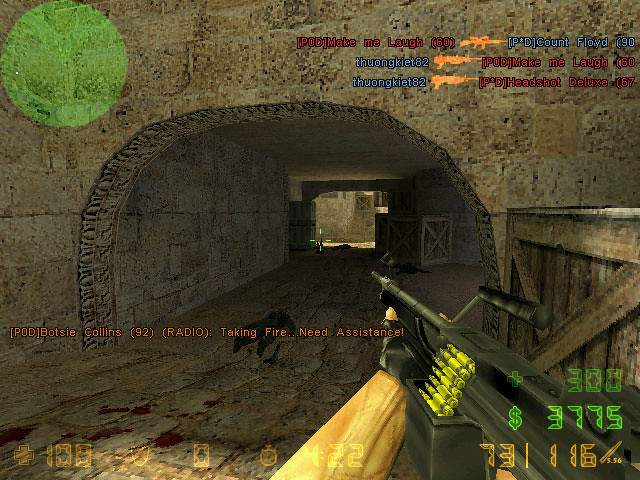This image is a detailed screenshot from a pixelated, retro-style first-person shooter video game. The UI elements are apparent, with a semi-transparent green circle map at the top left and a kill feed at the top right. The kill feed includes messages such as "Make Me Laugh, level 60, killed Count Floyd, level 90," and "Jungkeit82 killed Make Me Laugh and Headshot Deluxe." Player statistics are shown, with the money value at $3,775 and ammunition count at 116, displayed in the bottom right next to a money symbol. Health is indicated as 100 in the bottom left.

The in-game scene features the player's left arm, clad in a black glove, holding an assault rifle pointed down towards a stone underpass, revealing a tunnel-like structure adorned with a semi-circle entrance, stone walls, and floors. Just ahead, there is a crate and some boxes situated in the tunnel, which opens to a sunlit area on the other side. The immersive environment is enhanced with a chat message overlay that reads, "Botsy Collins Radio: Taking fire, need assistance." The browns and grays of the stone backdrop dominate the color palette of the scene, contributing to the gritty, old-school aesthetic of the game.